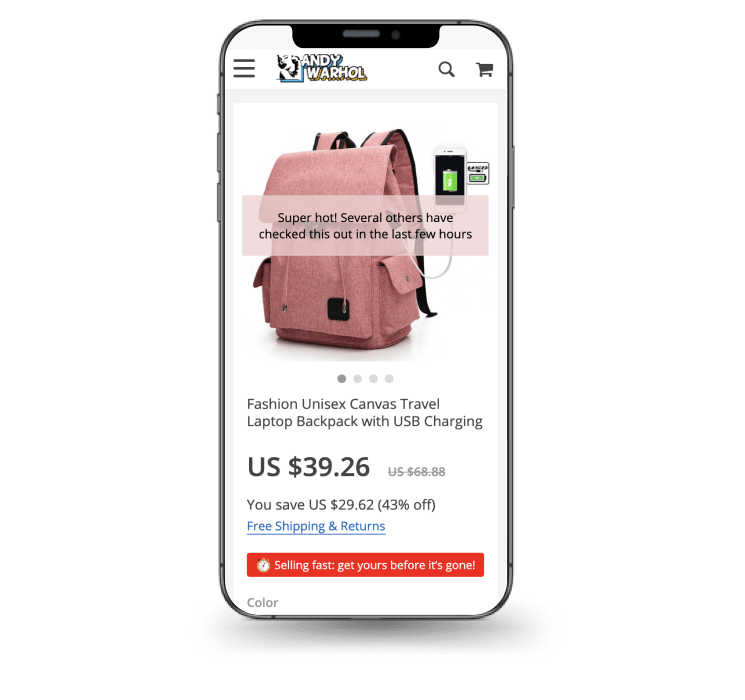Here is a cleaned-up and detailed caption for the described image:

---

The image showcases an iPhone in portrait mode, clearly delineating the device's outline. At the top of the iPhone screen, there are three horizontal lines representing a menu icon, followed by a logo and the text "Andy Warhol." To the right of this, there's a magnifying glass icon symbolizing search functionality and a shopping cart icon on the far right corner.

Below these icons, a product image is displayed prominently. The product is a pink book bag, equipped with a white wire extending from the bag, connecting to the iPhone. The iPhone's battery icon is shown with a light green fill and a white lightning symbol indicating charging. To the right of the battery icon, there's a partially illegible icon, possibly indicating another charging symbol or related text, though the resolution is insufficient for clarity.

An overlay of a light pink rectangle contains black text proclaiming "Super Hot." This text is accompanied by a note stating that "Several others have checked this out in the last few hours," and is followed by a sequence of ellipses. At the bottom of the screen, there are four ellipses, with the leftmost ellipse being a darker gray compared to the lighter gray of the others, indicating a page indicator.

The detailed product description reads, "Fashion Unisex Canvas Travel Laptop Bag with USB Charging Cable," priced at $39.26 USD. The original price of $68.88 USD is shown struck through in gray, highlighting a discount. The text emphasizes, "You save $29.62" (43% off), followed by an announcement in blue, underlined text: "Free shipping and returns."

Further down, enclosed in a rectangle with rounded corners, is an alarm clock icon next to the urgent message, "Get yours before it's gone!" Below this, the word "Color" is displayed in gray, but the rest of the text is truncated as it reaches the bottom edge of the screen.

---

This caption provides a comprehensive and clear visual description of the given image, emphasizing key elements and details.